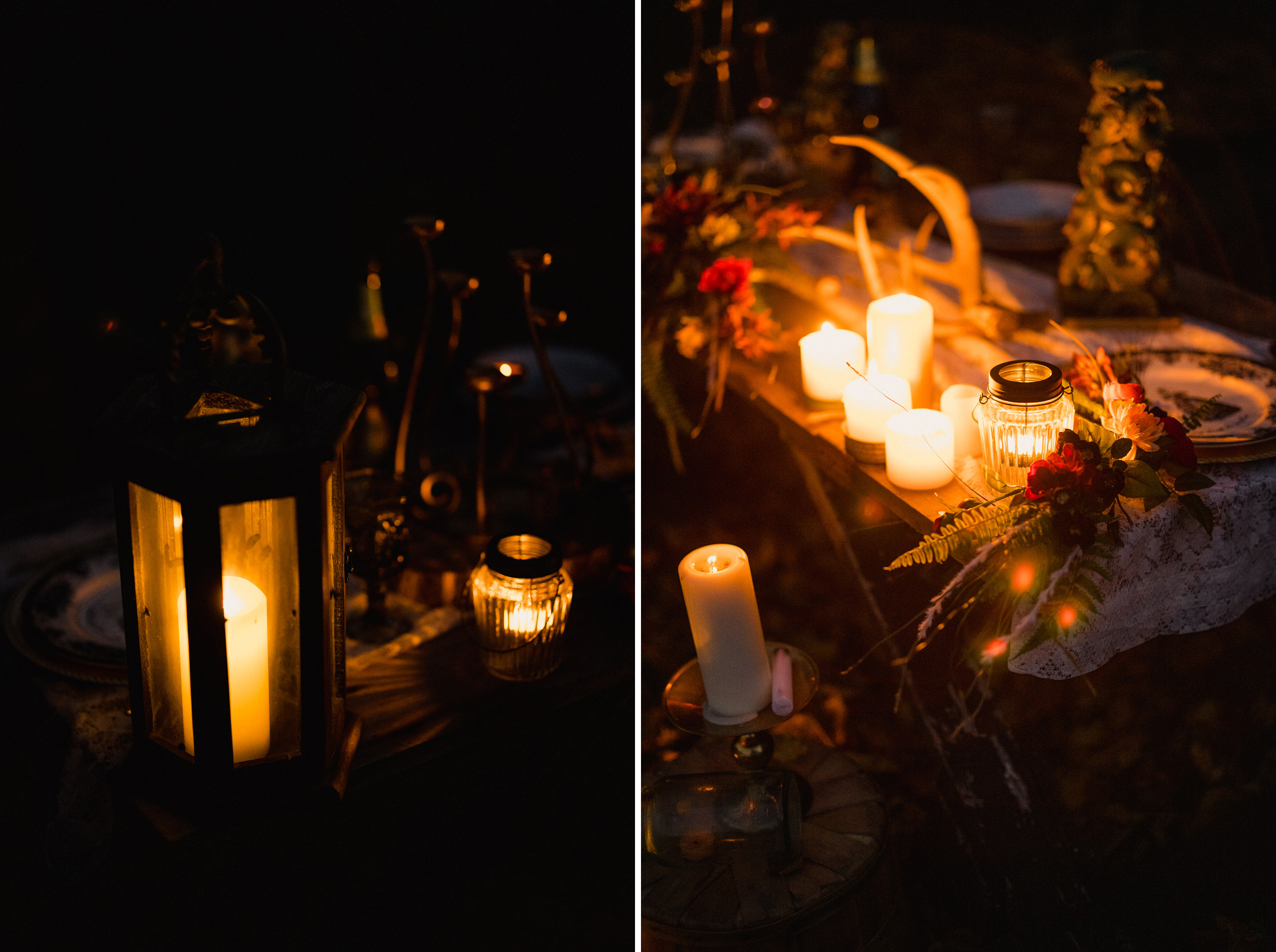This composite photograph features two images side by side divided by a white line. The image on the left displays a hexagon-shaped candle holder, black on the top and bottom, with bars on the sides and see-through glass encasing a lit, wine-colored candlestick. The candle emits an orangey glow, illuminating the dark setting. To the right of this is a smaller cylindrical candle holder with semi-refractive glass, further diffusing the orange light from the flame inside.

The image on the right showcases a brighter scene with multiple lit candles. Centrally, five candles with bright whitish-yellow flames rest on a shelf, with another candle beside them in a holder. Below these, there's a dimmer candle with a smaller, more orange flame. The background is adorned with red flowers placed on a brown wooden table, enhancing the outdoor nighttime ambiance shared in both images.